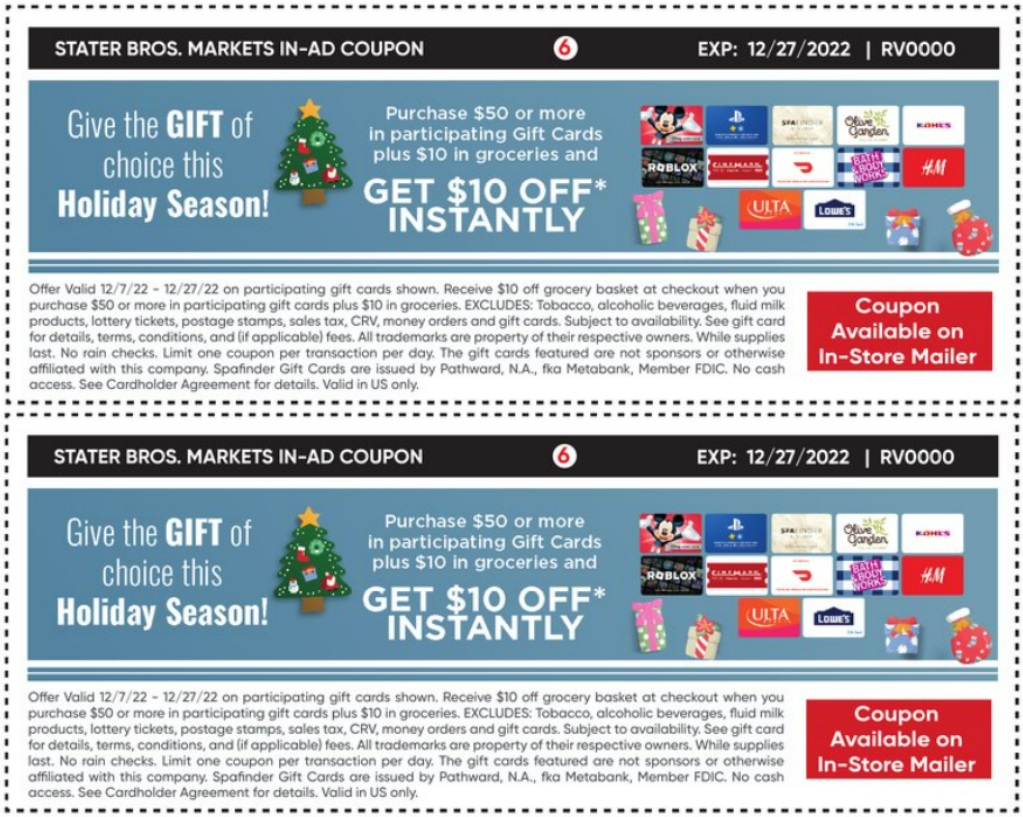In this image, we are looking at a detailed screenshot from a store's website, specifically from Stater Brothers Markets. The header of the image is in black with white text stating "Stater Brothers Markets In-Ad Coupon". A white circle with a red number "6" is visible, alongside the text "Expiration 12-27-2022 RV0000". Below this, a promotional message set against a blue background reads, "Give the gift of choice this holiday season," with the words "gift" and "holiday season" in bold white text. To the right of this message, there is an illustration of a Christmas tree adorned with decorations. 

The promotional offer, displayed prominently to the right of the tree, encourages customers to "Purchase $50 or more in participating gift cards, plus $10 in groceries, and get $10 off instantly". 

Further to the right, a selection of gift cards is showcased, including a Disney or Mickey Mouse card, followed by Roblox, Ulta, Lowe's, Olive Garden, DoorDash, Bath and Body Works, and H&M cards.